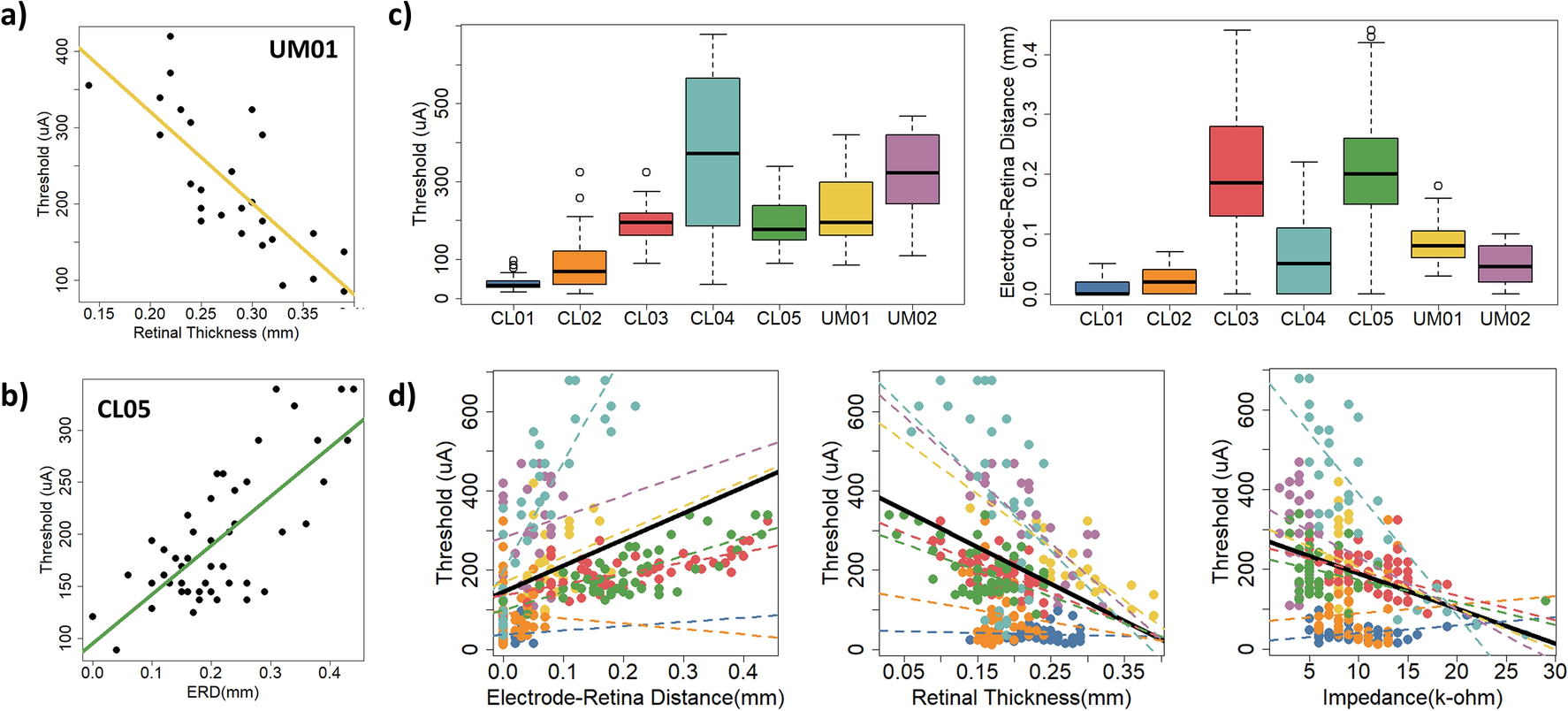The image is a detailed infographic featuring various types of scientific graphs and charts, divided into two rows. The top row consists of three illustrations: one square and two rectangular. The bottom row comprises four square illustrations. Each graph or chart is labeled sequentially from A to D, with three in the top row and four in the bottom row.

- **Top Row:**
  - **Graph A**: A square diagram showing retinal thickness, with a diagonal yellow line and scattered black dots. Measurements include thickness ranging from 0.15 to 0.35, and a threshold from 100 to 400 units (UA).
  - **Graph B**: A bar graph with colored bars labeled CL01 to CL04, showing various thresholds without thickness measurements.
  - **Graph C**: Another bar graph with different colors and labels, similar to Graph B in structure and detailing threshold levels.

- **Bottom Row:**
  - **Graph D**: This square graph, labeled B, features a green diagonal line and scattered black dots. The x-axis ranges from 0 to 4 millimeters and the threshold spans from 100 to 300 UA.
  - **Graph E**: An electrode-retina distance graph with colorful dots (green, red, orange, turquoise) and another set of measurements related to threshold and impedance in ohms, with ranges from 0 to 600 UA.
  - **Graph F & G**: Similar to Graph E, these contain various colorful dots and detailed measurements of electrode-retina distances and other scientific data points.

Overall, the infographic utilizes different colors and styles to represent detailed scientific data related to retinal thickness, thresholds, and impedance measurements in a clear and organized manner.